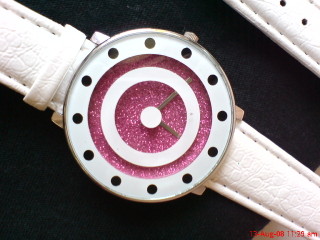The image portrays a wristwatch characterized by its striking and unique design. The watch has a white leather or faux leather band, visible on both the bottom and top right corners, suggesting the presence of an alternate or replacement band. The band features two black holes for fastening.

The round watch face is intricate, starting with a white metallic outer frame adorned with evenly spaced black dots that likely represent the hours at 12, 3, 6, and 9. Inside this frame is a concentric arrangement that alternates between white and glittery pink circles, creating a visually appealing spiral effect. The innermost circle is a white dot where the watch hands are attached. The watch hands themselves are silver with a white dot at their center connection point. 

The center of the watch face is a glittery pink section, adding a vibrant contrast to the surrounding white elements. The absence of traditional numbers is compensated by the strategic placement of dots, allowing viewers to approximate the time, which appears to be around 6:20. Despite this analog reading, a digital display at the bottom of the watch face indicates it is 11:29 a.m.